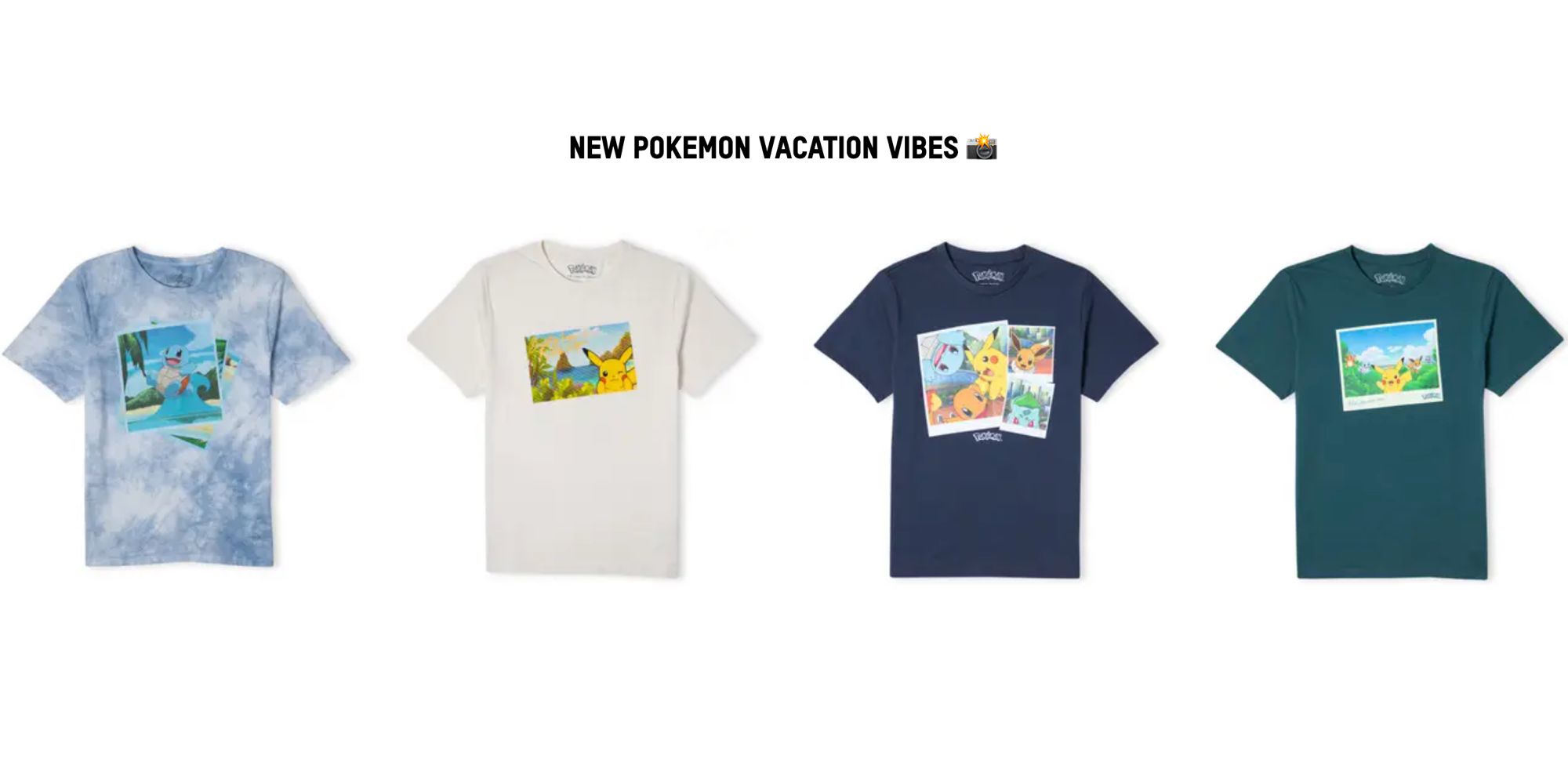The image features a collection of four short-sleeved t-shirts displayed against a plain white background. There are no outlines or boxes framing the image. At the top of the display, in bold black capital letters, the text reads "NEW POKEMON VACATION VIBES." To the right of this text, there is a small, indiscernible icon.

The t-shirts are arranged in a horizontal row. The first shirt is a light blue and white tie-dye pattern featuring a graphic on the front that appears to depict a beach scene with a Pokémon, although the details are too small to clearly distinguish. The second shirt is white and also contains a beach-themed graphic, possibly involving an ocean scene, but again, the specifics are too minute to be certain. 

The third t-shirt is navy blue and showcases three distinct images. Meanwhile, the fourth t-shirt is a dark teal green color and presents a graphic on the front that distinctly displays a blue sky with white clouds and green grass.